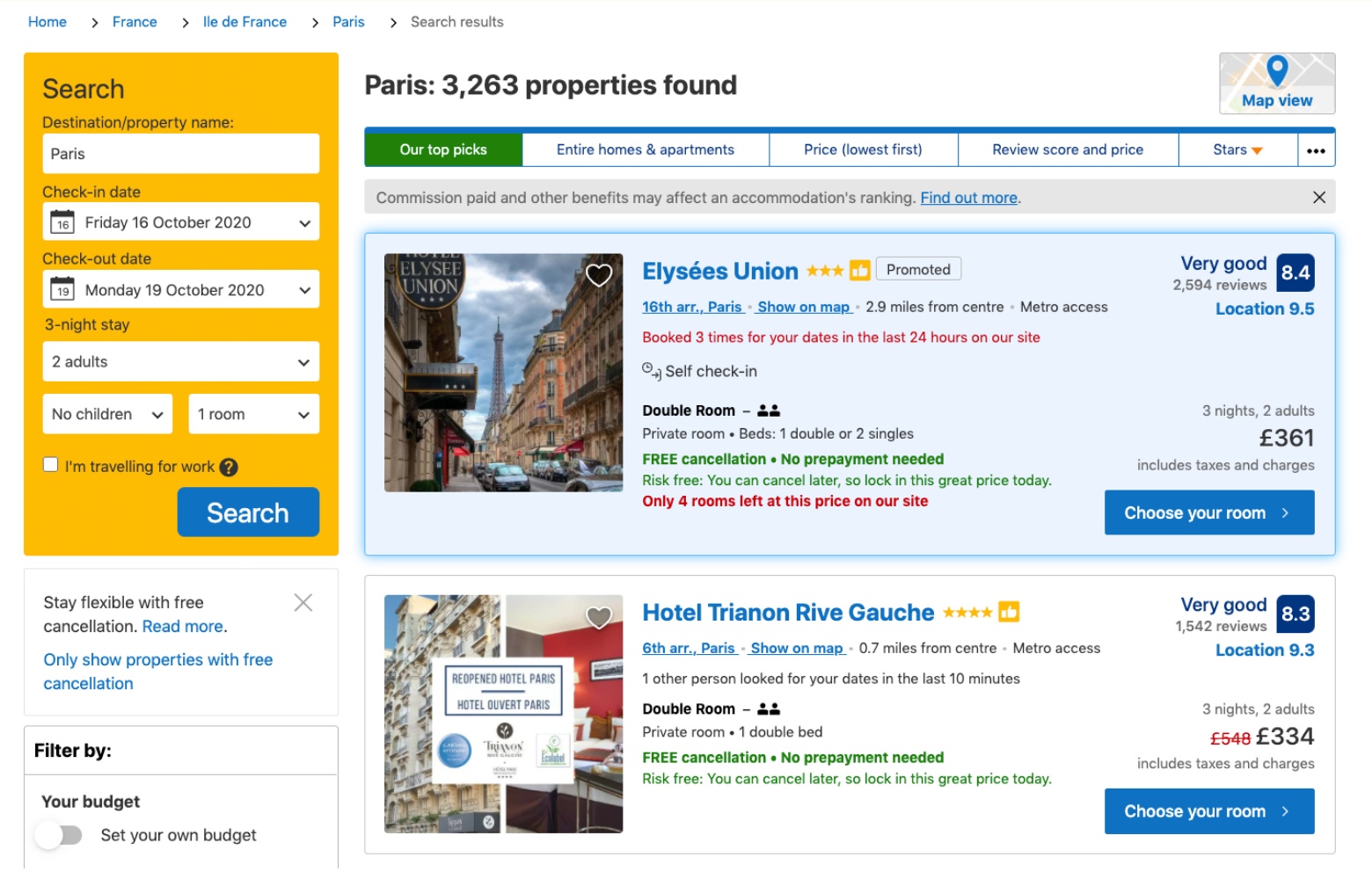Screenshot of a travel booking website interface. The top navigation bar features a white background with blue font, displaying tabs labeled "Home," "France," "La France," "Paris," and in gray, "Search Results." On the left side, there's an orange box with "Search" written in black. Below this, entry fields prompt for "Destination/Property Name," populated with "Paris." The "Check-in Date" is selected as "Friday, 16 October 2020" and "Check-out Date" as "Monday, 19 October 2020," indicating a three-night stay. Details mention "two adults," "no children," and "one room."

A blue button with white text displays "Search." Below, in black, it says "Stay flexible with free cancellation" and in blue, "Read more." Further down, another blue option reads "Only show properties with free cancellation." A section in black notes, "Fail to fit your budget? Set your own budget."

At the top part of the results area, it states in black "Paris, 3,263 properties found." Various filter tabs are present: the active one is green with white text "Our Top Picks," followed by white-background boxes with blue text "Entire Homes and Apartments," "Price (Lowest First)," "Review Score and Price," and "Stars." At the bottom, two properties are listed: "Ulysses Union" and "Hotel Tryon and Rye Gulch."